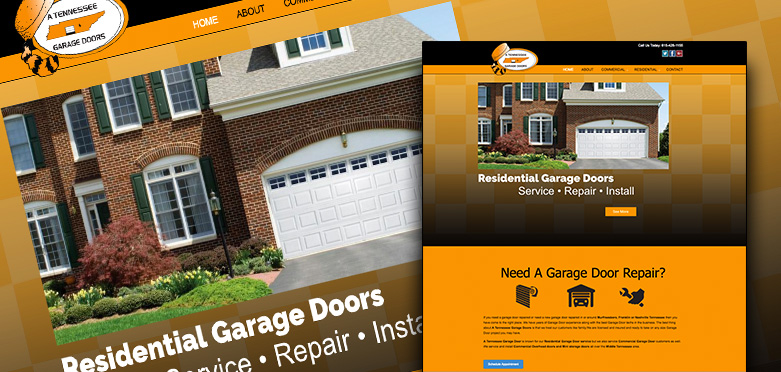A professionally composed advertisement photograph is set against an orangish-beige background, featuring promotional materials for "Tennessee Garage Doors." Dominating the image is a large, two-story brick home showcasing a pristine white garage door adorned with decorative windows along the top. This focal point illustrates the high-quality residential garage door services provided. 

Amidst the scene, two flyers introduce additional details. The primary flyer, slightly askew, reveals sections of the company’s website with partial views of navigation tabs like "Home" and "About." Denoted at the bottom of this flyer are the services offered: "Residential Garage Door Service, Repair, Install." 

Adjacent to the main flyer is a smaller advertisement set against an orange backdrop, with bold black text that inquires, "Need a Garage Door Repair?" The smaller ad features a series of miniature images including paper towels, a garage with a car inside and the door halfway up, and a hand gripping a wrench signifying repair services. The meticulous composition and color scheme emphasize the company’s dedication to professional and comprehensive garage door solutions.